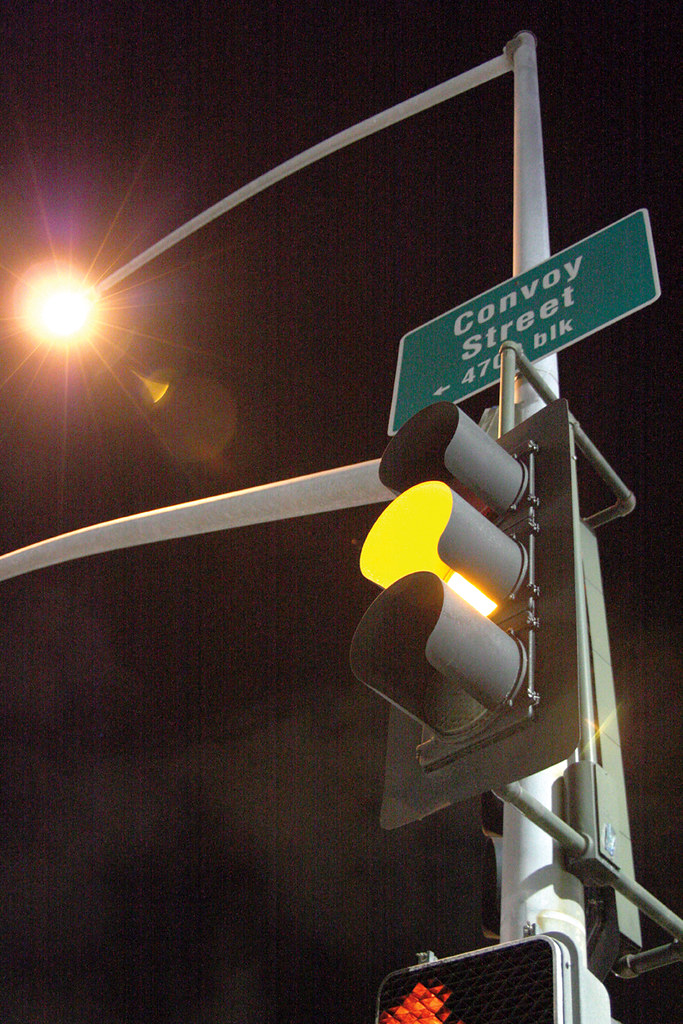This nighttime photograph captures a ground-up perspective focusing on a streetlight and a traffic signal. The scene is enveloped in darkness, with the black void of the night sky as the backdrop. The prominent feature is the streetlight, mounted on a sizeable silver-gray boom arm that glows under the artificial light. Affixed to this streetlight post is a green directional sign, clearly marked with "Convoy Street" and an arrow pointing left, accompanied by the partially legible text "470" and "BLK."

In parallel with the streetlight, the stoplight features illuminated signals. The central yellow light in the triad of the stoplight is lit, casting a warm hue. Below the stoplight, a pedestrian walk signal is partially visible, its top half emanating a glowing orange light, adding a hint of urban life to the scene. The convergence of streetlight, traffic signals, and signage creates a complex yet captivating composition against the night’s inky canvas.